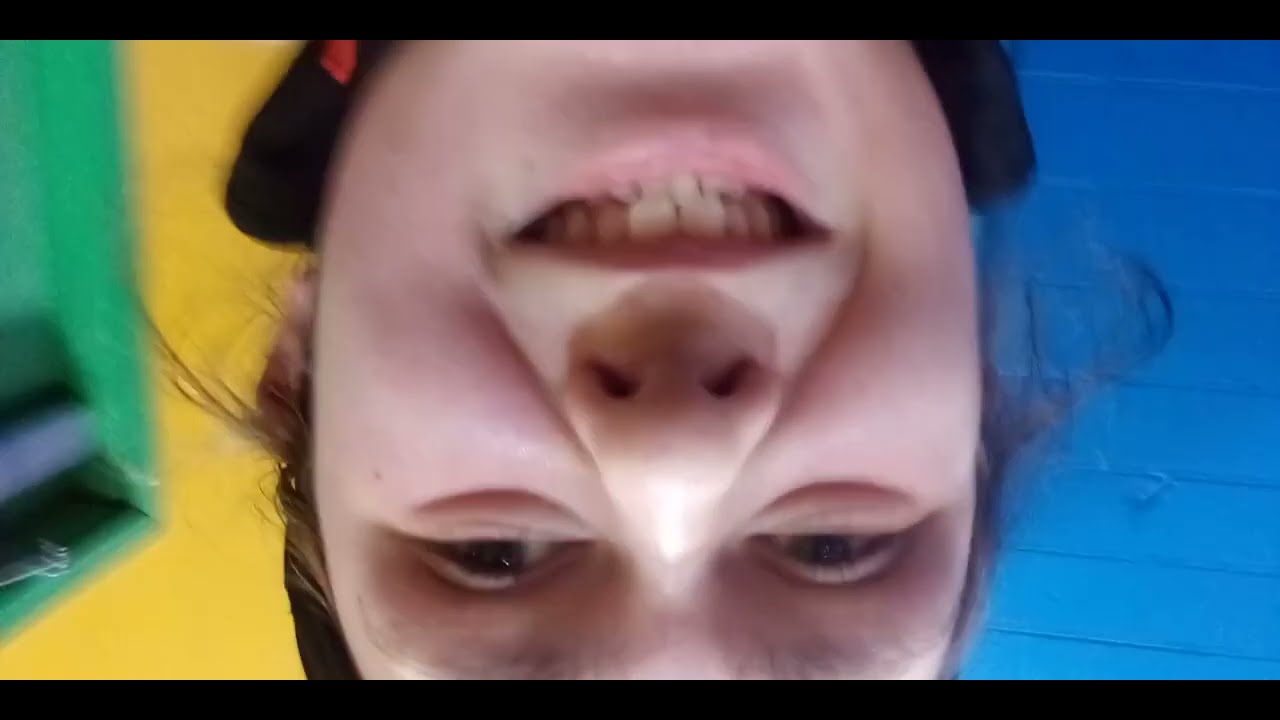The image is an upside-down picture of a smiling female with short brown hair. She is possibly wearing a black hat with her hair peeking out slightly. Her teeth are visible, though slightly yellow. The background features a blue and yellow wall, with vertical blue boards on the right and a green doorway or closet on the left. There's also a red object on her jacket. The overall image appears blurry and is framed within a high-definition television screen, bordered by narrow black bands at the top and bottom.